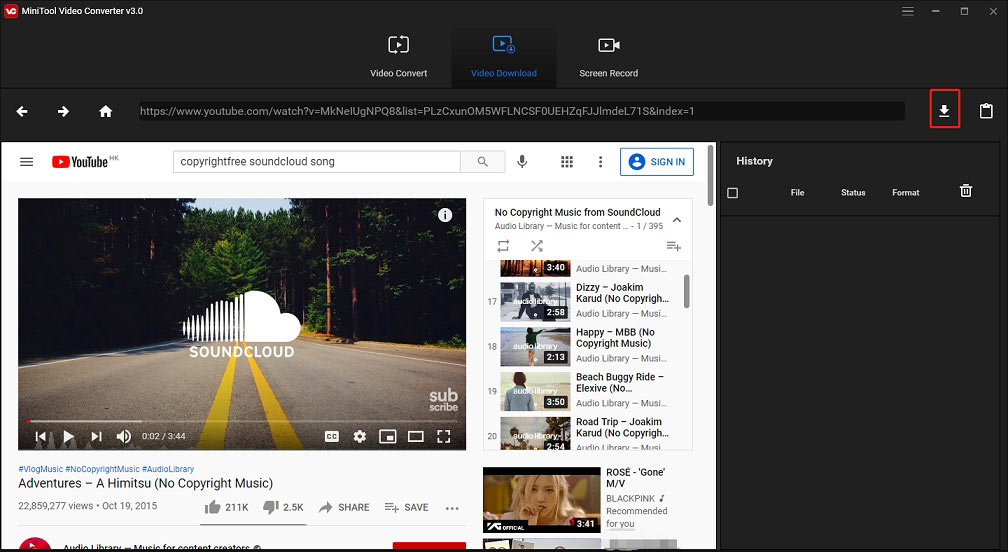This image features a digital interface primarily dominated by a black background. Centrally, there appears to be a video player or converter labeled with "video content," along with additional options such as "view" and "record." In the upper-left corner, a small red icon is visible, although its details are obscured.

Towards the right side of the image, a YouTube pop-up promotes a copyright-free song from SoundCloud. This section includes a thumbnail depicting a scenic road flanked by forests, titled "Adventures." Above this, the familiar SoundCloud icon, shaped like a cloud, is prominently displayed.

The right-hand column of the interface showcases a list of other non-copyright music tracks from SoundCloud. The largest thumbnail in this list features a girl identified as "Rosie." Further up the column, additional thumbnails represent other tracks, each accompanied by photographs that presumably relate to the respective songs. The entire design is framed by a red box around the download icon, drawing focus to the interactive elements of the interface.